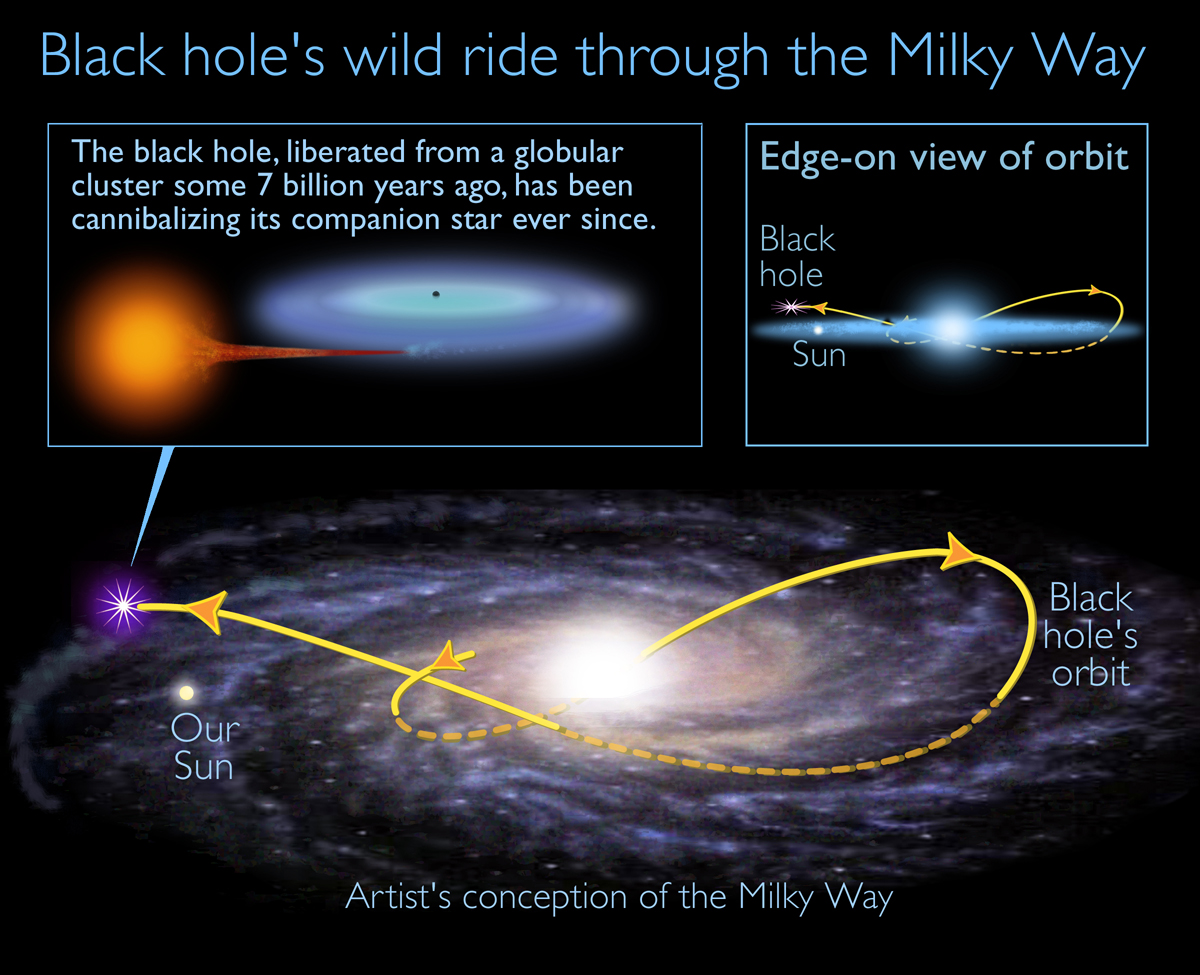This detailed illustration depicts a black hole's complex journey through the Milky Way. The main focal point is a yellow, lopsided infinity sign that signifies the orbit of the black hole relative to our Sun's position in the galaxy. Above the main image, a blue heading reads "Black Hole's Wild Ride Through the Milky Way." Below the heading, the illustration is divided into three sections, each outlined in blue on a black background.

On the left, a rectangular box contains a cross-sectional view of the Milky Way, showing the orbit of the black hole and the Sun. Within this section, a yellow arrow loops asymmetrically around the galaxy, emphasizing the path of the black hole.

To the right, another detailed diagram highlights the black hole's origin and destructive behavior. It reads, "Black hole liberated from a globular cluster some 7 billion years ago and has been cannibalizing its companion star ever since." This box features a disc representing the event horizon of the black hole, a bluish spiral indicating the accretion disk, and a red-orange sphere depicting the companion star being gradually consumed, with streaks of stellar material extending toward the black hole.

Below these two primary sections, an "Artist's Conception of the Milky Way" is labeled, illustrating the larger galactic structure. A yellow dot marks the location of our Sun, while yellow orbital arrows highlight the black hole's path throughout the galaxy. The meticulous details combine to create a comprehensive view of the black hole's trajectory and impact within the Milky Way.